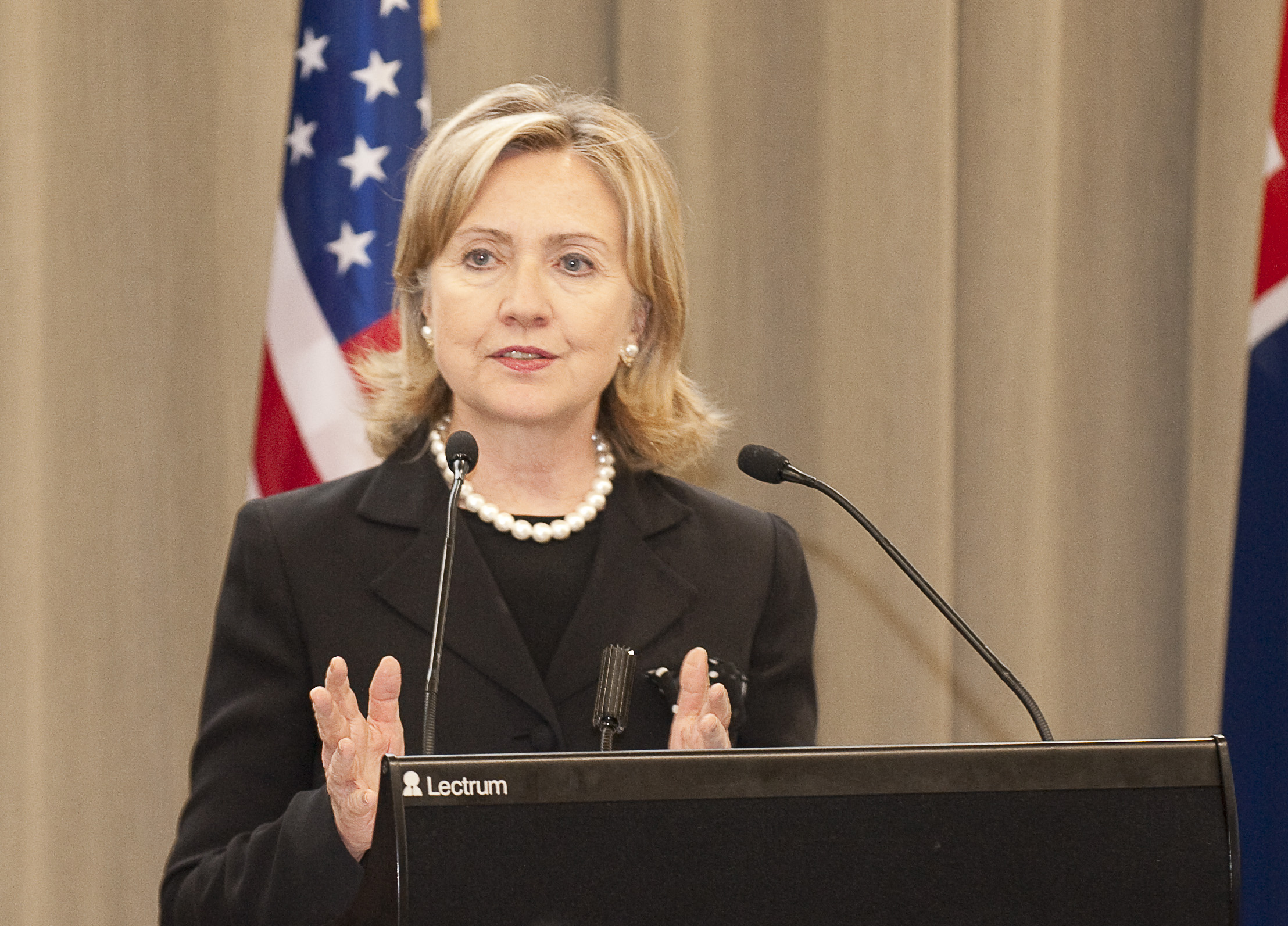This photograph captures Hillary Clinton standing at a black podium adorned with three microphones, two of which are tall and positioned at chin level, while a shorter one sits in the center. Clinton, identifiable by her blonde hair that falls to her neck, is dressed in a black blazer with shoulder pads over a black undershirt, and she is wearing a white pearl necklace. The background consists of tan, light brownish curtains, and features two flags: an American flag to her left, and another indistinguishable flag to her right, showing only red, white, and blue colors at the edge. The podium itself is plain, except for the word "lectrum" in white letters on the top left, accompanied by a small image of a person. Clinton appears to be in the midst of delivering a speech or address. The setting is indoors, with the overall color scheme comprising tan, red, white, blue, yellow, and black tones.